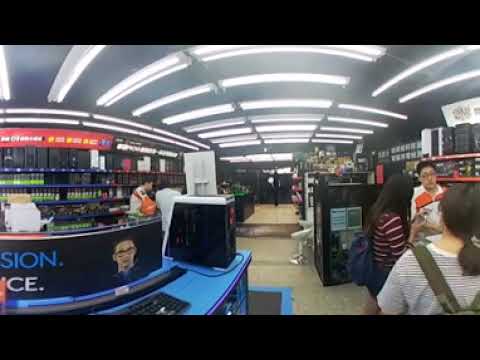The picture appears to be taken inside a store, potentially a school supply or an electronic store, but there are indications it might also be an alcohol or a bookstore. The setting includes aisles and numerous shelves filled with various items, some possibly in fancy black boxes similar to wine packaging. To the left, there's a blue desk or counter with a computer setup, including a CPU and a keyboard, possibly indicating a checkout or service terminal.

In the bottom right corner, three younger individuals, likely students due to their backpacks, gather. The closest to the camera is a young woman with dark hair in a ponytail, wearing a striped shirt and a backpack. Next to her is another woman in a red and pink striped shirt, also with a backpack. To the right of them, a young man with dark hair and glasses is seen in an orange and white shirt. 

The ceiling is lined with numerous fluorescent lights, providing bright illumination throughout the store. The overall image is slightly blurry and has a warped effect, suggesting it might have been taken with 360-degree imaging, making it challenging to discern finer details.